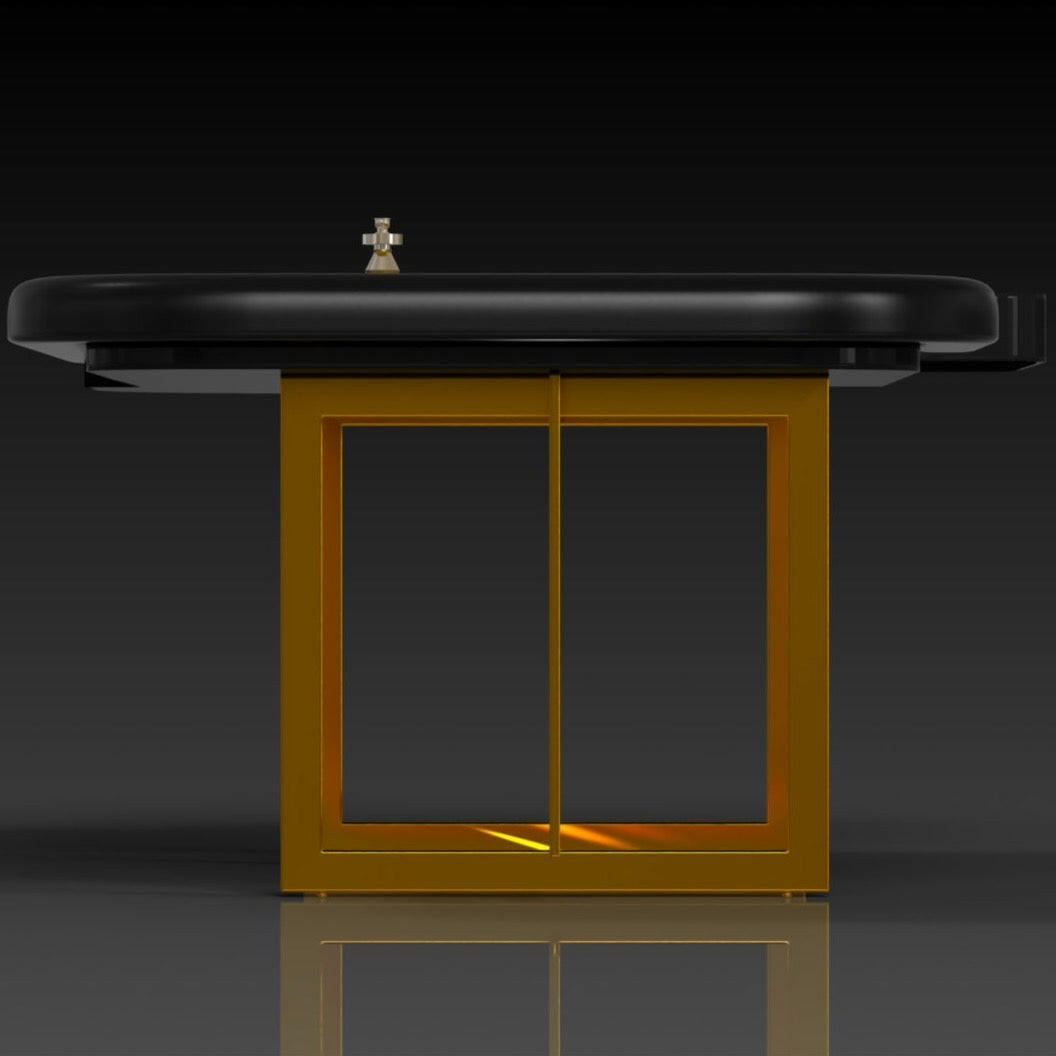In this intricate computer-generated image, a striking piece of art or furniture is prominently displayed. The base of the structure resembles a golden window frame with a horizontal gold line running through its center. The stand emanates a reflective glow, indicating a light source shining upon it. Atop the base sits a black surface, which seems to be a tabletop, possibly cushioned, akin to what one might find in a doctor’s office. This dark surface is complemented by a metal element on the right, resembling a knob or handle, suggesting it might be interactive. At the center of attention on the black top is a silver cross statue. The overall scene is captured in a grayish ambiance, fading to black at the top, with the highly polished floor mirroring the golden base. The backdrop appears to be a dark, reflective expanse, enhancing the mysterious and modern aesthetic of the image.